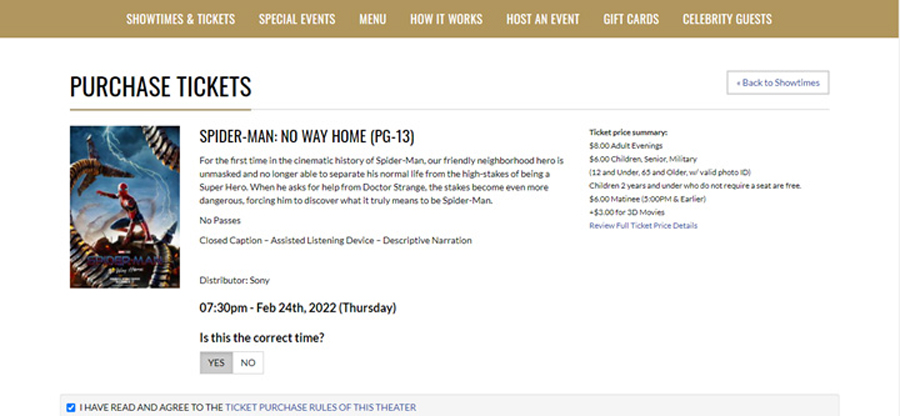## Detailed Caption for the Provided Image:

The image showcases a webpage from a ticket purchasing website, specifically designed for buying movie tickets. The page features a gold backdrop with white text. At the top, there are several navigation options listed: "Showtime and Tickets," "Special Events," "Menu," "How It Works," "Host an Event," "Gift Cards," and "Celebrity Guests."

Central to the page is a prominent section titled "Purchase Tickets." Below this header is a picture of Spider-Man accompanied by a poster for the movie "Spider-Man: No Way Home," rated PG-13. The poster includes a short synopsis: 

"For the first time in the cinematic history of Spider-Man, our friendly neighborhood hero is unmasked and no longer able to separate his normal life from the high stakes of being a superhero. When he asks for help from Dr. Strange, the stakes become even more dangerous, forcing him to discover what it truly means to be Spider-Man." A note indicates that no passes are accepted for this film.

The accessibility features listed include closed captioning, assistive listening devices, and descriptive narration. Additionally, the distributor of the film is identified as Sony.

The ticket details feature a specific showing time of 7:30 p.m. on Thursday, February 24, 2022. The selection is confirmed with a checkbox indicating this is the correct time. At the bottom of the page, there is a statement that reads, "I have read and agreed to the ticket purchase rules of this theater," which requires acknowledgment.

On the right-hand side, there is a price summary section displaying the ticket prices: $8 for an adult evening ticket and $6 for children, seniors, and military personnel. There is also a note about photo ID requirements and a mention that children under 12 who do not occupy a seat are admitted for free.